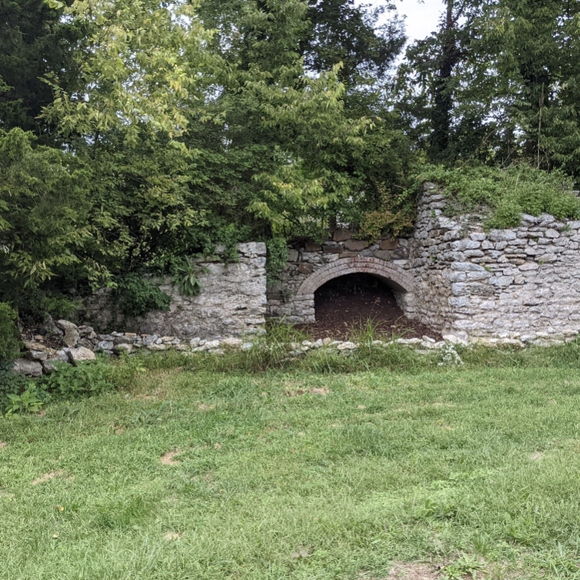This realistic square photograph captures an outdoor scene during a slightly overcast day with a bluish-white sky. The setting appears to be a wild, unkempt field in a forested area, dominated by abundant greenery. The foreground features uneven, lush grass, leading to a prominent stone structure in the center of the image. This man-made stonework, likely an old bridge, drain, or tunnel, consists of a substantial cobblestone wall about 10-15 feet tall, embedded into a grassy hillside. The wall has a low, arching opening at its base, approximately 6 feet wide and 3 feet high, suggesting it might have once served as a vent, cellar entrance, or water passage. The archway is now partially filled with dirt, adding to the archaic and mysterious feel of the structure. Surrounding the stone feature are dense trees and shrubs, framing the main subject of the photograph. Additionally, a foot-high wall runs along the front of this intriguing formation, further defining the scene.